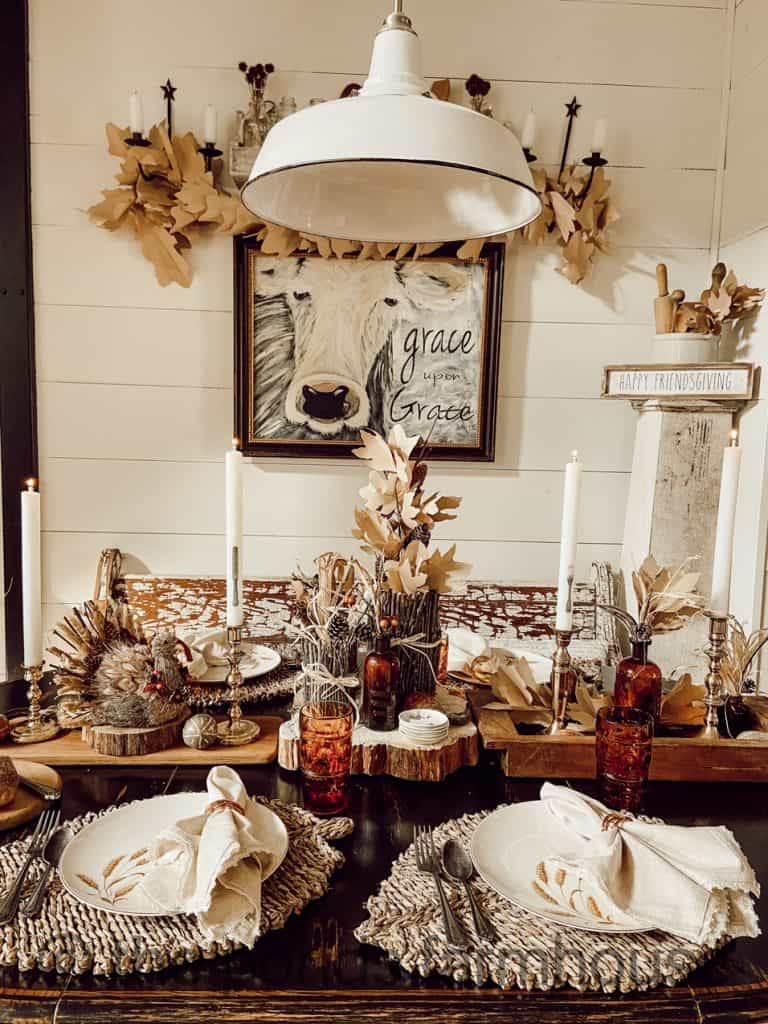The image presents a meticulously arranged tablescape that exudes an autumnal, Thanksgiving ambiance. Dominating the arrangement is a table adorned with white circular plates, atop which sit neatly folded napkins and stalks of wheat, suggestive of the fall harvest. The glasses on the table have a distinct brown tint, enhancing the earthy, seasonal vibe. A centerpiece of artificial leaves and a faux turkey perched on a brown wooden log further underscore the Thanksgiving theme. Gold candle holders with white candles imbue the scene with elegance, complementing the festive decor. 

The surrounding room adds to the overall narrative, with white walls featuring horizontal lines and a prominent painting of a horse, labeled "Grace upon Grace," in a brown frame. Above the painting, candle stands embellished with brown leaves create a cohesive flow from the decor on the wall to the table setup. A white spherical lamp dangles from the ceiling, providing soft illumination. A sign at the corner reads "Happy Friendsgiving," confirming the occasion's celebratory nature. The attention to detail extends to table mats, well-placed utensils, bottles, and various decorative items, crafting a warm and inviting festive environment.